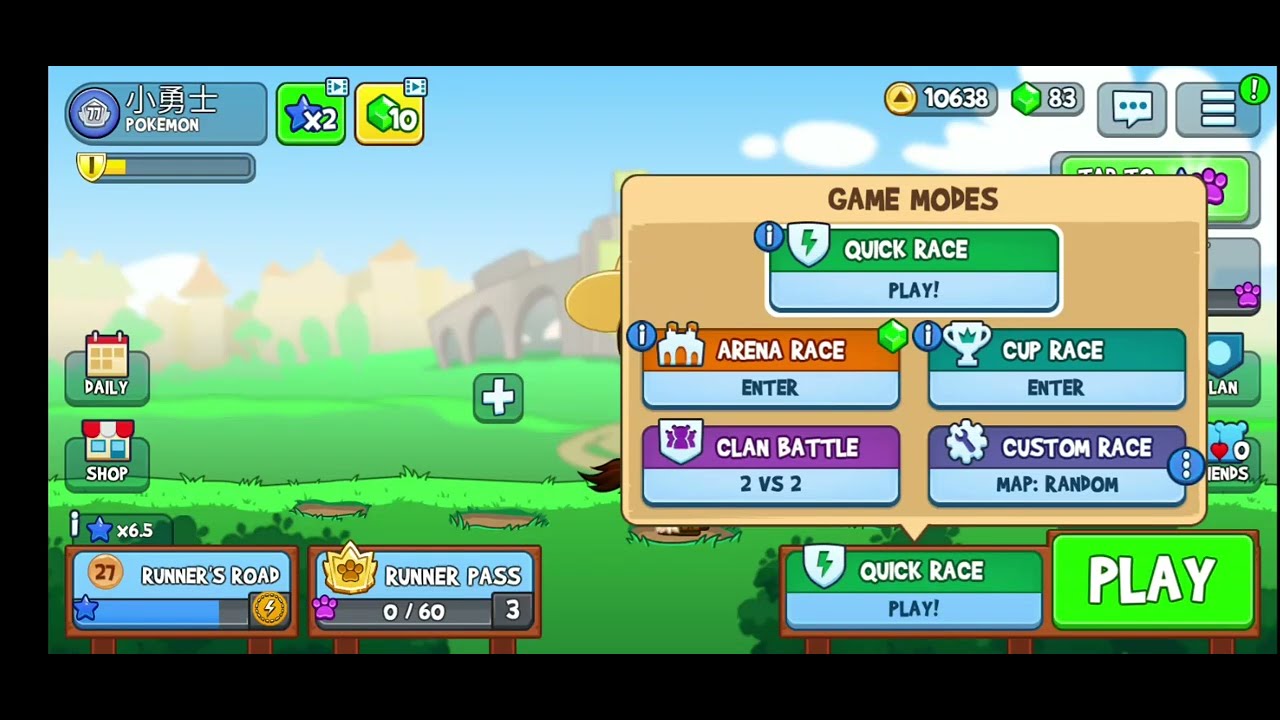This image is a detailed screenshot from a Pokemon video game that showcases various gameplay elements and user interface features. The backdrop features a vibrant sky with blue hues and white clouds, a light gray building in the center, and some orange buildings further left in the distance. In the upper left corner, there is a Pokemon character alongside text that says “Pokemon” in both English and Asian characters. Just below this, a blue logo displays the number 77, with a yellow status bar indicating energy levels next to it. 

To the right, a green logo with a blue star displays "x2," and a yellow box with a green square shows the number 10. The upper right section of the screen contains several status bars and icons, including an orange circle with a triangle that says 10638, a green square with the number 83, a sky blue message icon with three dots, a hamburger menu icon, and a green circle with an exclamation mark.

The right-hand side of the screen features a beige pop-up box titled "Game Modes," displaying various options such as Quick Race, Arena Race (Enter), Cup Race (Enter), Clan Battle, 2 vs. 2, Custom Race, and Map Random. Each of these modes is highlighted with unique color schemes. 

In the bottom left corner, there are small wooden signposts labeled "Runner's Road" and "Runner's Pass 0/60." Additionally, another quick race section appears with a green play button labeled "Play" in white letters. Throughout the image, there are various green, blue, and orange icons and text elements providing additional data and gameplay information. The very top and bottom of the image, as well as the left-hand side, are bordered by a black background that frames the game's interface elements.